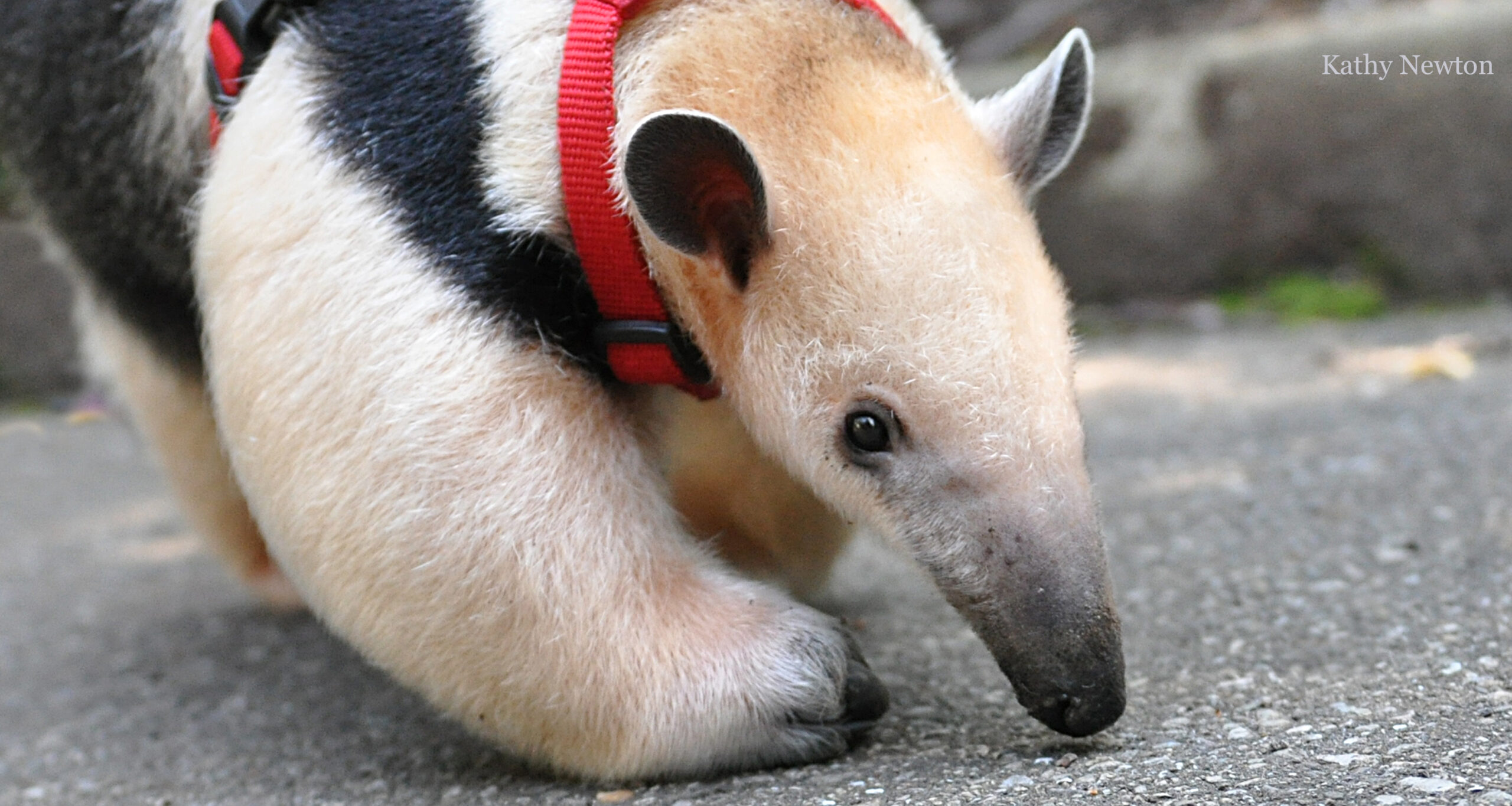This detailed photograph captures a Southern Tamandua, an animal with distinct features resembling both an aardvark and an anteater. The Southern Tamandua sports a fur pattern that includes a tan back and arms, interspersed with black sections, particularly noticeable as black spots on its back and the sides of its arms. It has round black eyes, a long snout, and ears that are dark inside. The tips of its feet and paws are black, adding to its unique appearance. A red leash with a black buckle is attached to the Tamandua, suggesting it may be in a controlled environment, possibly a zoo. The animal appears to be sniffing the ground, which is gray in color, likely asphalt. The background of the image is blurred, but patches of green and gray can be seen, with some rocks and grass at the bottom. In the top right corner of the image, the name Kathy Newton is written in white, possibly indicating the photographer or a caption.